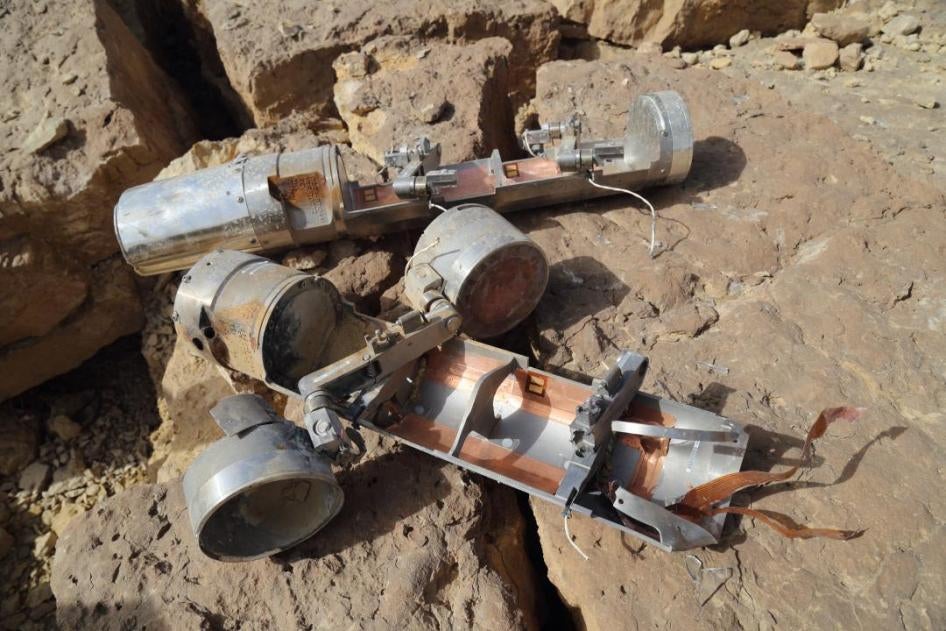The image depicts a desolate, rocky terrain that appears to be a desert-like environment, with gray or brown rocks scattered across the ground. Toward the center, there are two large cylindrical tubes, each approximately a foot long and four to five inches in diameter, that are broken and dismantled. The tubes, which have silver bases, are dusty and slightly rusty, with metal pieces and wires protruding from their broken sections. They appear to have been exposed to the elements for some time, as indicated by their weathered condition. The tubes are resting on and over the cracks in the rocks, casting shadows. There are visible orange connectors attached to parts of the equipment, suggesting they were once part of a more complex structure. While the exact nature of the cylinders is unclear, they resemble time capsules or components of an improvised explosive device (IED), though there are no signs of explosive residue or damage around them.